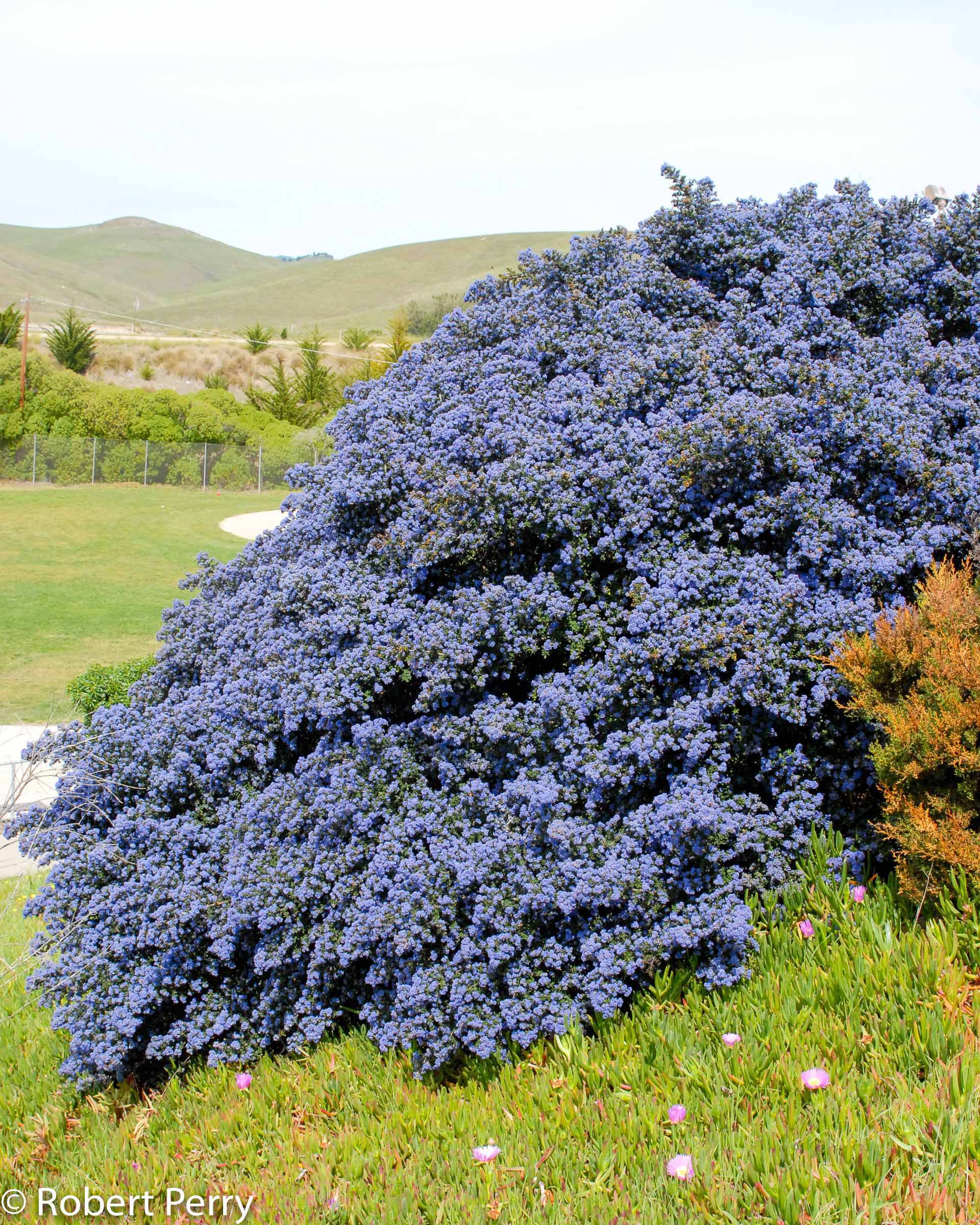The photograph, taken by Robert Perry according to the copyright in the bottom left corner, captures a vibrant and detailed landscape. The focal point is a large, interconnected bush dominating the center and right side of the image, covered in tight clusters of bluish-purple flowers, resembling lavender. The bush is lush and overgrown, sprawling across the foreground where shorter green grass and small pink flowers peek through. On the right, there is a small section of what could be a dying orange-brown plant or another type of bush. The background reveals neatly maintained lawns suggesting a possible golf course, with two small sandy spots visible on the top left. A chain-link fence runs beyond the grassy area, leading to patches of trees and rolling hills that gradually turn mountainous in the hazy distance. The sky is a light blue with little to no cloud coverage, contributing to the bright, clear atmosphere of this daytime scene.